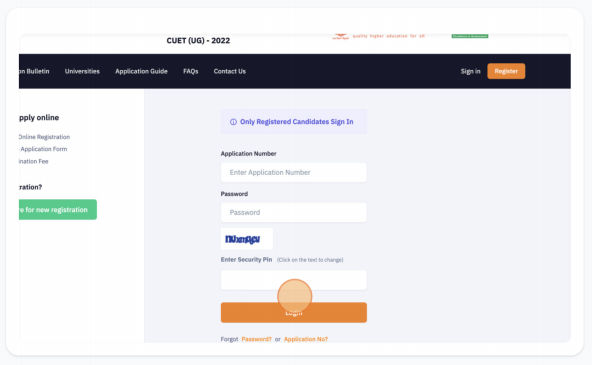The image features a webpage related to an application process, prominently titled "CUET (UG) 2022" at the top. To the right of the title, there is some barely readable orange text followed by a green bar. Below this section is a black navigation bar with the following options from left to right: "Bulletin," "Universities," "Application Guide," "FAQs," and "Contact Us." On the right end of this bar, there is a "Sign In" option accompanied by an adjacent orange button labeled "Register."

Further down the page, a blue prompt states "Only Registered Candidates Sign In." Below this, there are input fields for users: "Application Number" in black text with a white input field labeled "Enter Application Number," "Password" with an empty space labeled "Password," and a "Security Pin" feature in blue text. The security pin is a distorted jumble of letters, and the instruction "Enter Security Pin, click on the text to change" is displayed alongside a white box. Below these fields, an orange circle is visible, and an orange-red button labeled "Login." Underneath this section, there is a "Forgot Password or Application Number" link.

On the left side of the page, there are additional links labeled "Apply Online," "Online Registration," and "Application Form," with a green button situated below these options.